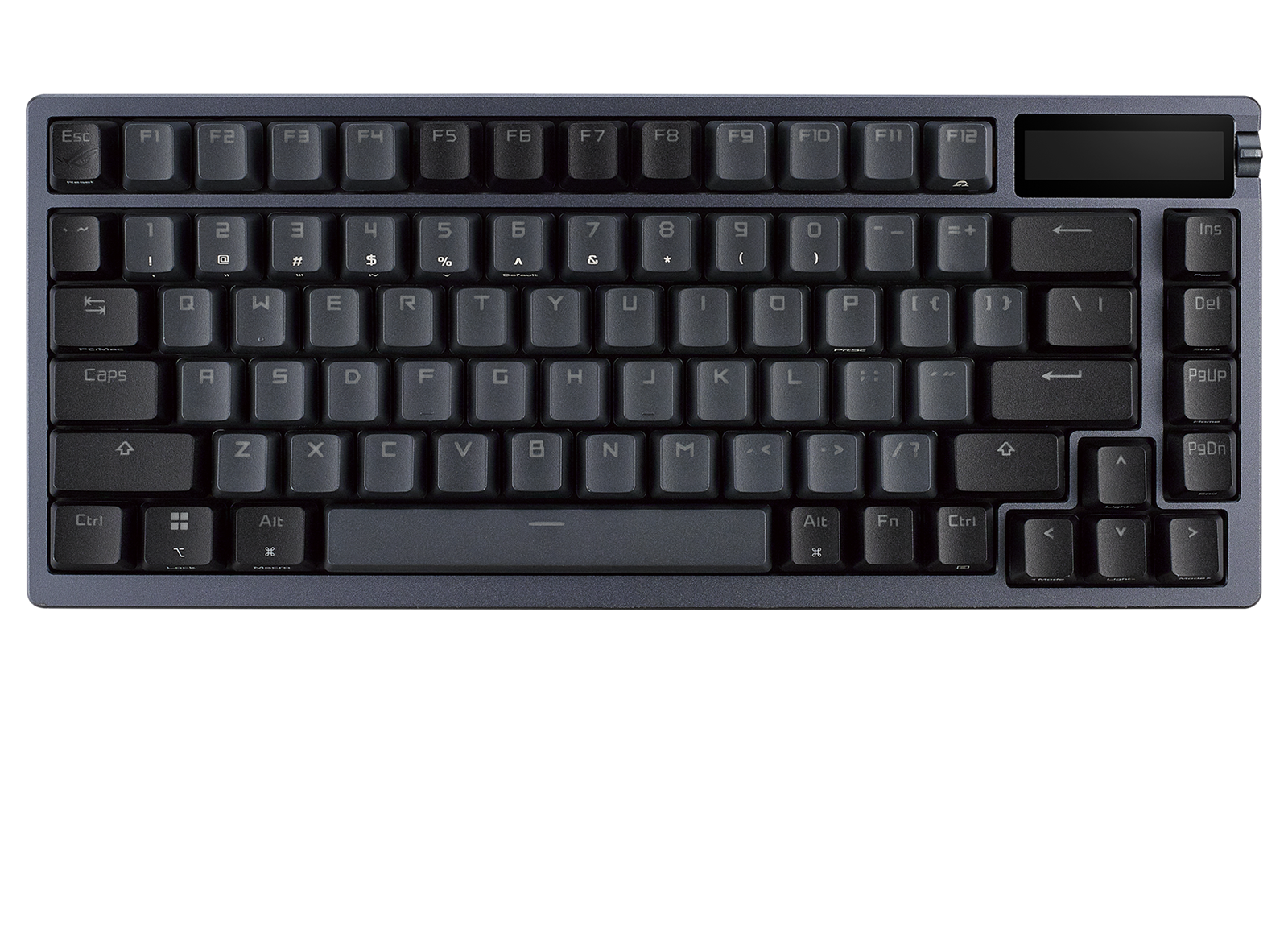This is a detailed photograph of a compact, black mechanical keyboard set against a white background. The keyboard's frame is shaped as a slightly rounded rectangle, creating a minimalistic aesthetic. It omits a keypad on the side and instead features a compact layout with tightly nestled keys. 

The top row of keys includes specialized function keys, starting with ESC followed by F1 through F12, which are distinctly bright white with additional symbols in gray. Below this row is a line of number keys, and further down lies the standard QWERTY layout for the alphabet in five subsequent rows. To the right, the keyboard hosts navigation keys such as Insert, Delete, Page Up, and Page Down, with the arrow keys positioned at the bottom of this section.

The text on the main keys is a light gray, suggesting some wear and tear, especially on the heavily used letters, which indicates the keyboard has seen regular use. A curious small feature or screen is visible at the top right corner of the keyboard, next to which lies a trim of plastic encasing the function keys area. The design elements combine to make this a modern, efficient keyboard typical for computer use.